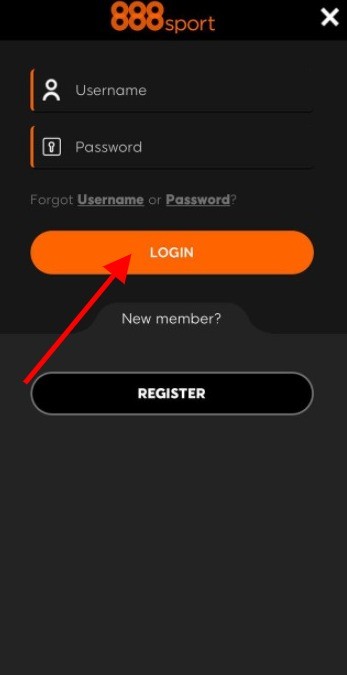The image is a portrait-mode screenshot with a predominantly black background. At the top center, the logo "888 Sport" is prominently displayed in a bright orange color. The top right corner features a white 'X', likely for closing the screen or dialog. 

Beneath the logo is a form section for user login. This form includes text fields for "Username" and "Password," each flanked by vertical orange stripes. Below these fields are live links for "Forgot username or password" underlined and clickable.

A large orange button labeled "Login" sits below the text fields, emphasized by a big red arrow pointing towards it. The text on this button is orange on orange, making it difficult to read.

At the bottom of the form, against a lighter black background, the text "New Member?" appears in white. Adjacent to this text is a big black button with white bold letters, easier to read, saying "Register." This button has ample black space around the text. 

Overall, the visual elements guide users to either register as a new member or log in with existing credentials by following the red arrow to the "Login" button.